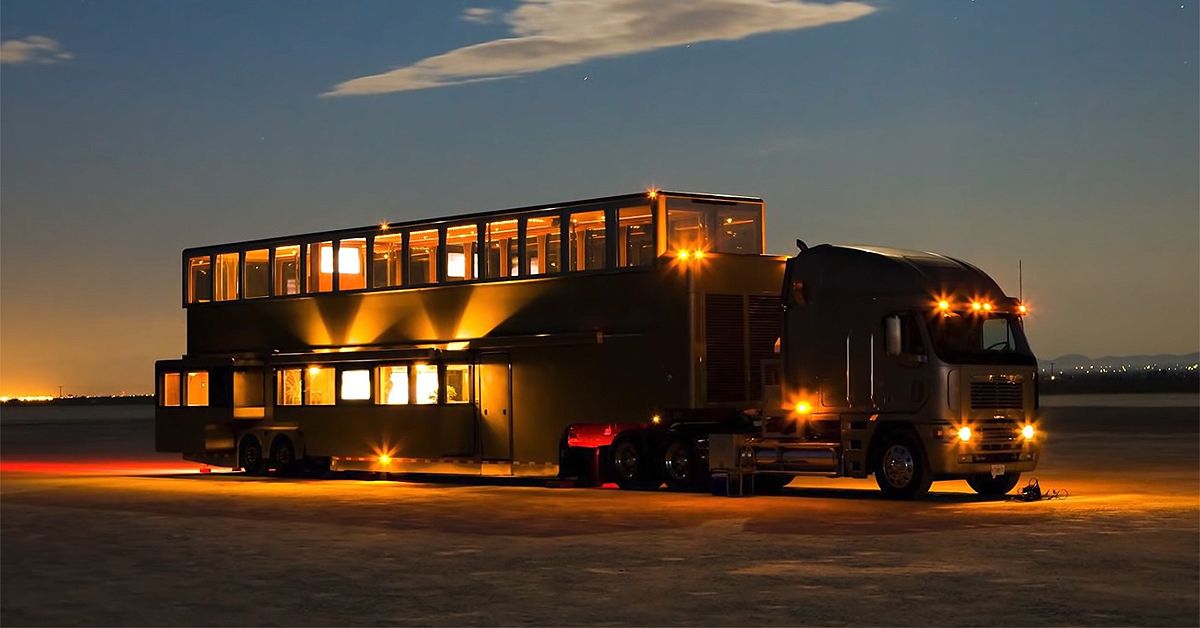In this color photograph taken in the evening, a large, black truck is prominently featured, parked in an open, flat area that appears to be an empty parking lot. The truck is equipped with vibrant orange headlights and adorned with numerous lights, casting a glowing yellow and red hue on the ground around it. The sky, a deepening blue with hues of orange from the setting sun, is dotted with white clouds and a few visible stars. Attached to the truck is a unique, modified trailer that has been transformed into a two-story structure resembling an upscale RV, tiny house, or even a mini mobile hotel, featuring extensive glass windows that dominate its facade. In the background, the lights of a distant cityscape and the silhouette of mountains add depth to the scene, enhancing the luxurious and adventurous aura of this impressive mobile dwelling.